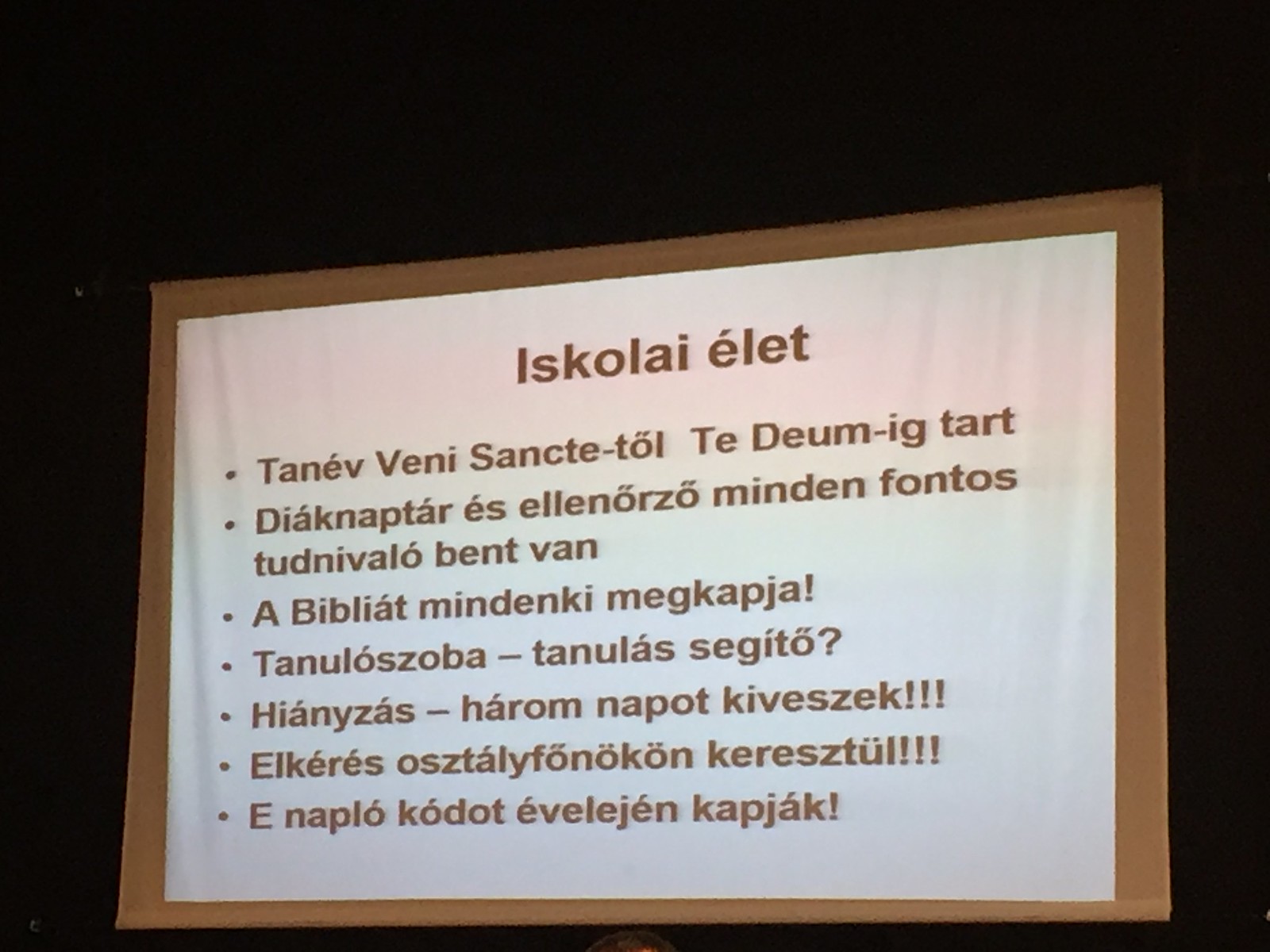The image features a framed document against a solid black background, possibly cropped to create this effect. The document appears to be a set of seven school life rules written in Hungarian and is presented in a landscape format on what looks like a linen-textured piece of paper. The text is in a plain, Arial-like font, and the frame has a wooden appearance. At the top of the document, in the center, the words "Iskola Élet" are displayed in brown font, indicating "School Life." The bulleted rules address various aspects of the school schedule, including the beginning and end of the school year, and the obligation to read from the Bible, suggesting it may be for a Catholic school. The detailed elements of the text have been translated to convey specifics about the academic calendar and important regulations for students. Each rule line elaborates additional crucial points, contributing to the comprehensive guideline structure of the document.